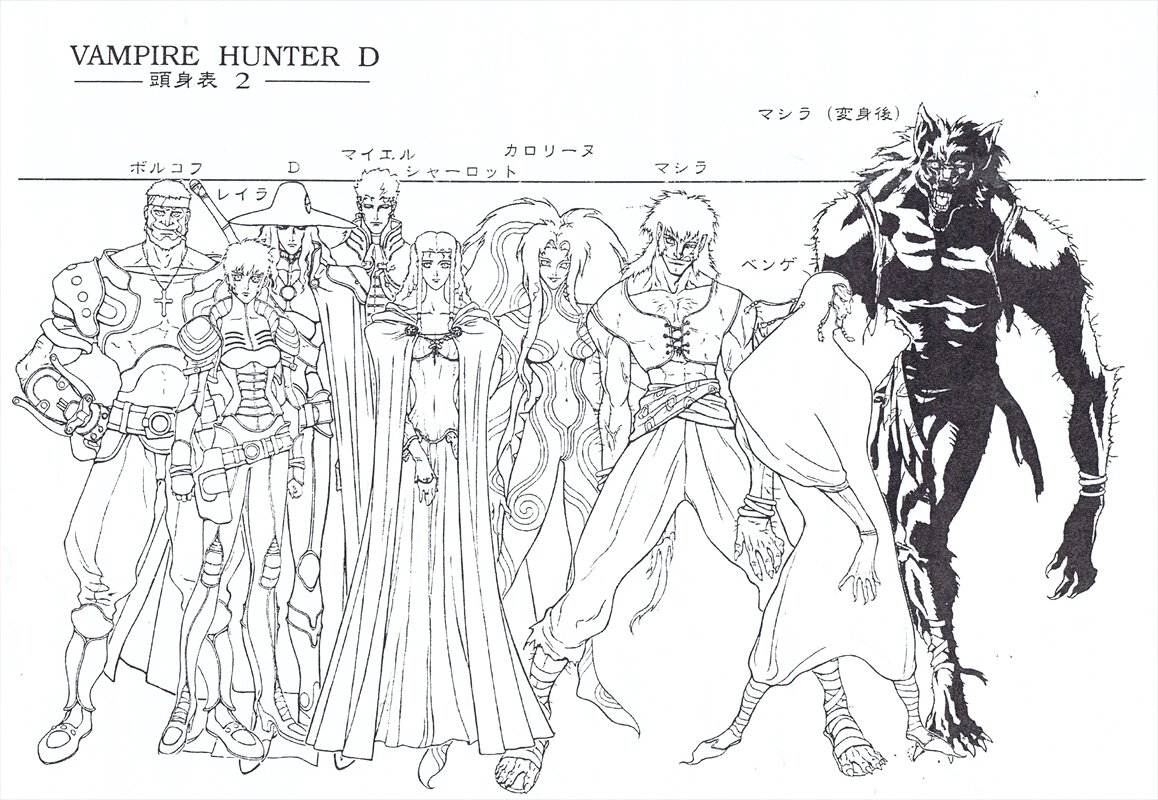In this black and white illustration, which seems to be concept art from a DVD for "Vampire Hunter D" with text in Japanese above the individual character concepts, we see an array of detailed cartoon characters, both human and non-human, all facing forward. Starting from the left, there is a strong-looking man wearing armor, a headband, and a cross necklace. He is followed by a woman in a superhero-like armor suit, slightly shorter than him. Next, a mystical figure labeled with the letter D, characterized by a long-brim hat and flowing hair, reminiscent of a witch with a wide, large collar, stands prominently. Following this figure is another tall man, though his clothes are less visible, he appears to be adorned with a significant, wide collar. To his right stands a royalty-like figure, draped in long, flowing clothes and possessing long hair. Adjacent to her is a woman adorned in a form-fitting suit with intricate swirly patterns and large, voluminous hair. Beside her stands a large, muscular man with clothing that hints at a Hulk-like influence. Finally, to the far right is a towering, wolf-like character, distinguished by its upright stance, long arms, taloned fingers, and taloned toes. The diversity and intricate detailing of each character highlight their unique attributes and roles within the narrative.